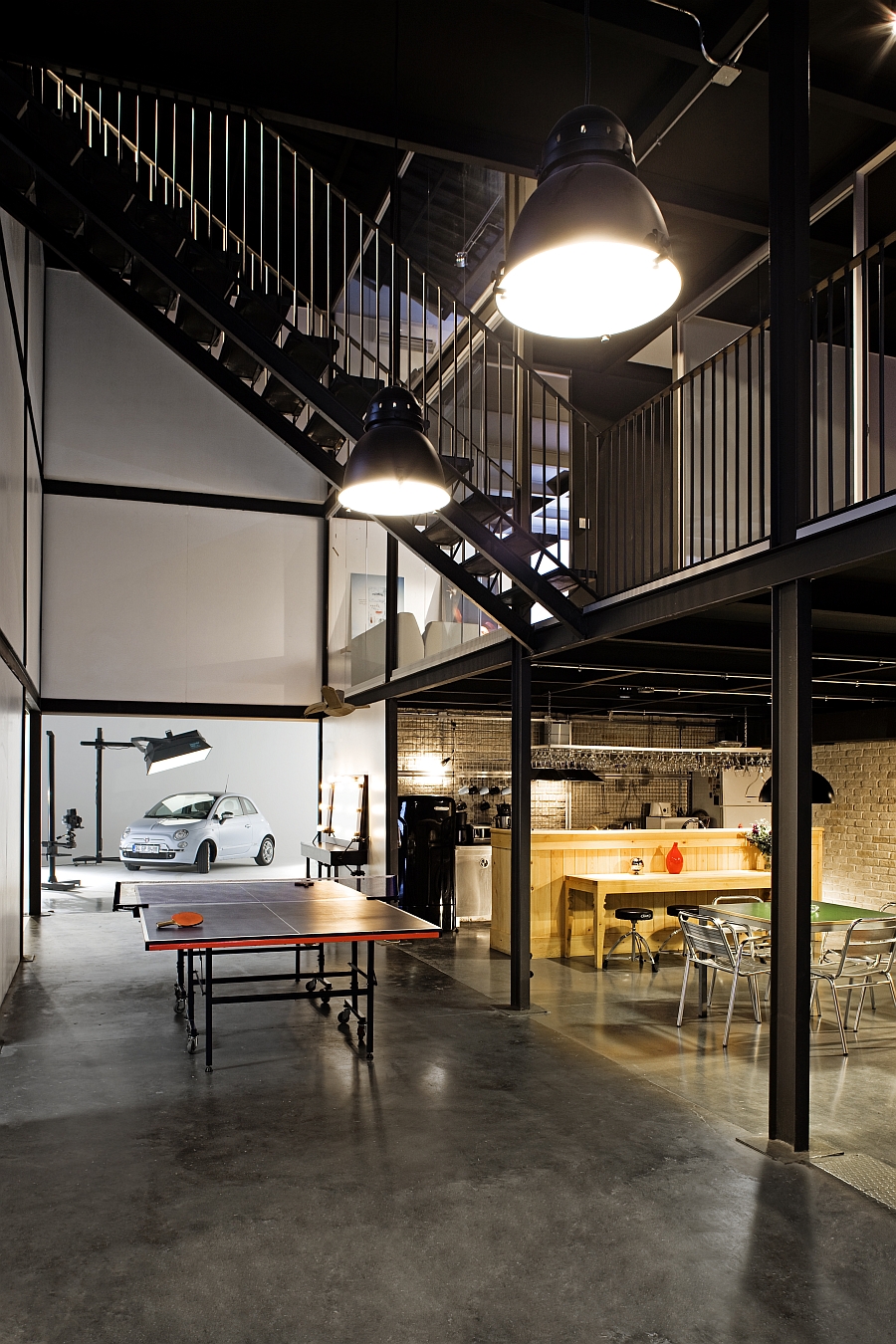The image captures a spacious, multi-story indoor setting that likely serves as a converted warehouse, now functioning as a home or versatile studio. The scene is dominated by a palette of black, white, gray, orange, brown, and silver. The setting features high ceilings adorned with large light fixtures and white panels trimmed in black, enhancing the expansive feel.

On the left side, a kitchenette area sits below the lofted upper floors, equipped with a wooden bar, a refrigerator, and other appliances. A small table with simple folding lawn chairs adds a casual touch, while a green dinette table with chairs adds a splash of color. A ping-pong table is set up to the right, suggesting recreational use.

Near the back of the room, a tiny economical car rests under a large, photo-studio-like light, with a makeup vanity mirror positioned nearby, hinting at a potential photography or showroom space. The background includes both a metal table and chairs and an upstairs area accessible by a wrought iron black staircase. This upper level features a balcony with glass panels that enclose a cozy living space with a couch and possibly some artwork.

The overall layout suggests a multifunctional environment blending residential, recreational, and possibly professional uses, all within the industrial charm of a repurposed warehouse.